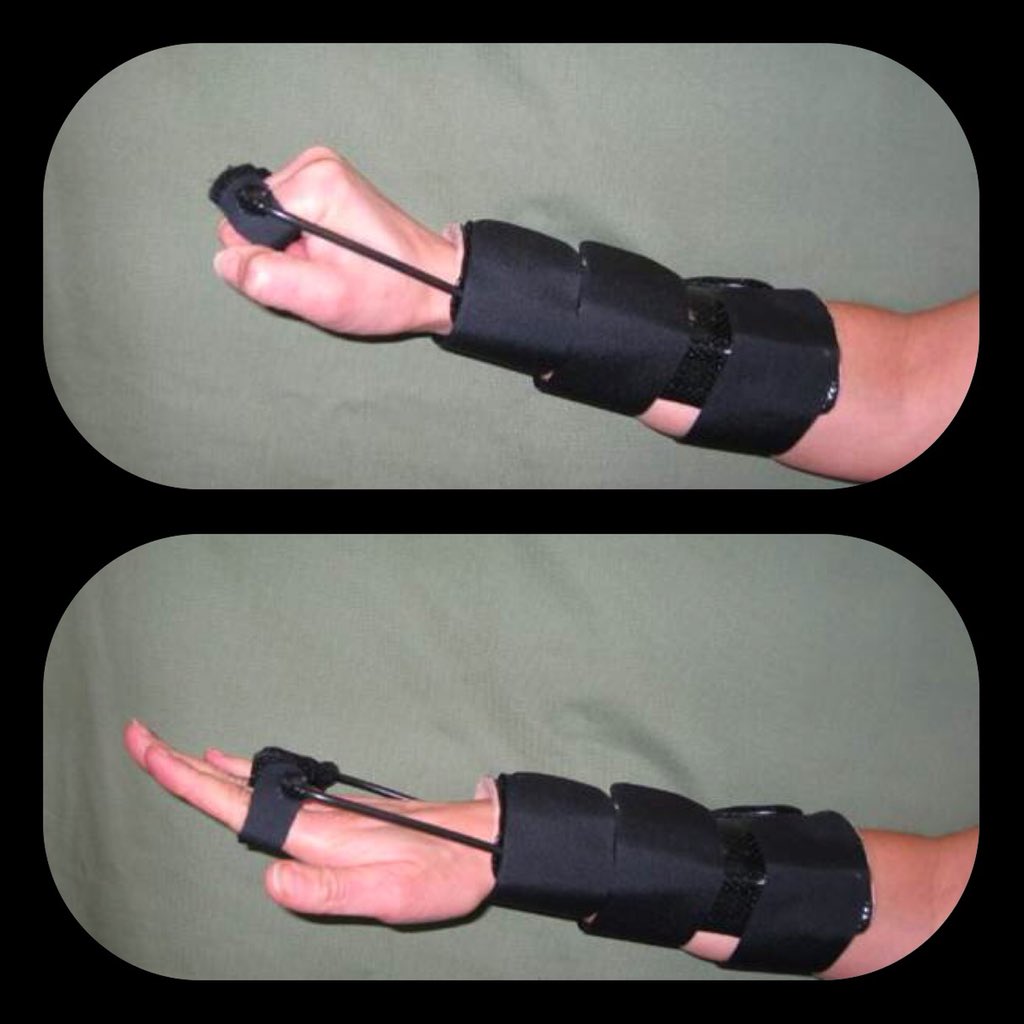The image shows two photographs, one above the other, of a man's hand and forearm. Both photos feature a black rehabilitation or exercise apparatus. The top photograph, set against a gray background with rounded rectangular edges and a black outer border, shows the arm extending from the right side with the thumb facing the camera, knuckles up. The hand is closed into a fist. The apparatus includes a wrist guard that extends almost to the elbow and is secured by three adjustable Velcro straps around the forearm. Additional components of the device extend from the wrist to a strap that wraps around the fingers.

In the bottom photograph, set against a similar gray background, the same arm is positioned with the fingers extended straight out to the left, and the thumb once again facing the camera. This image highlights the full extension of the fingers and more of the apparatus's structure, including the additional strap connected to the fingers. The purpose of the contraption seems to be for either strengthening or rehabilitating the hand and forearm by facilitating repetitive fist-clenching and finger-stretching exercises.